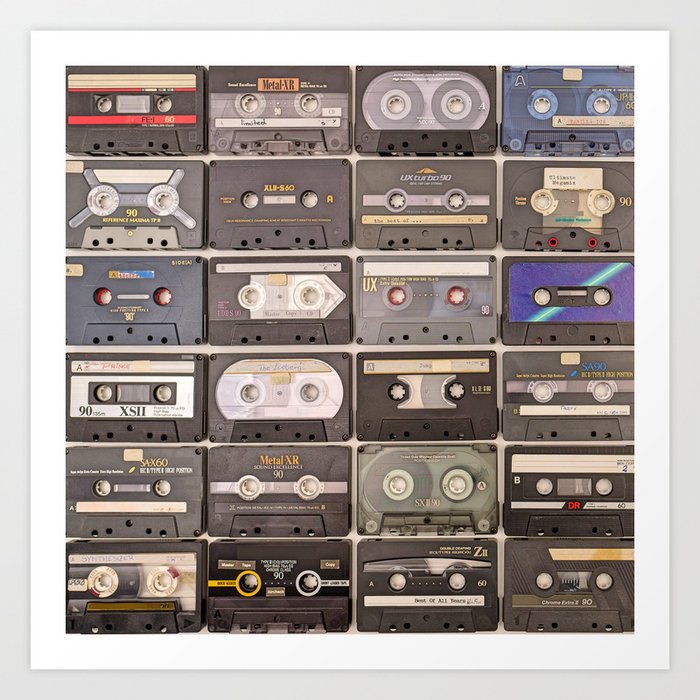The photograph captures a collection of 24 audio cassette tapes arranged in a meticulous grid on a light-colored surface. Organized into six rows and four columns, each tape is laid flat and closely spaced, creating a visually appealing pattern. In the top left corner, a black cassette tape features striking red stripes on its label. Adjacent to it is a clear tape with a prominent black stripe at the top, followed by a black tape with a clear middle section revealing the spools of ribbon, and a clear blue tape at the far right. The second row starts with another black tape that has clear lines radiating from each side of the holes, transitioning to a mix of black and grey tapes, many with distinctive labels such as "FE-160," "Metal XR," "90 Reference Maxima IP2," and "UX Turbo 90." The third row highlights tapes with labels that include designs reminiscent of cameras or binoculars. The bottom rows feature a diversity of tapes, including dark and chrome blacks, various shades of grey, and notable patterns like a galaxy style and camouflage. Across all rows, the tapes exhibit diverse branding and playback positions, adding to the rich tapestry of this nostalgic collection.